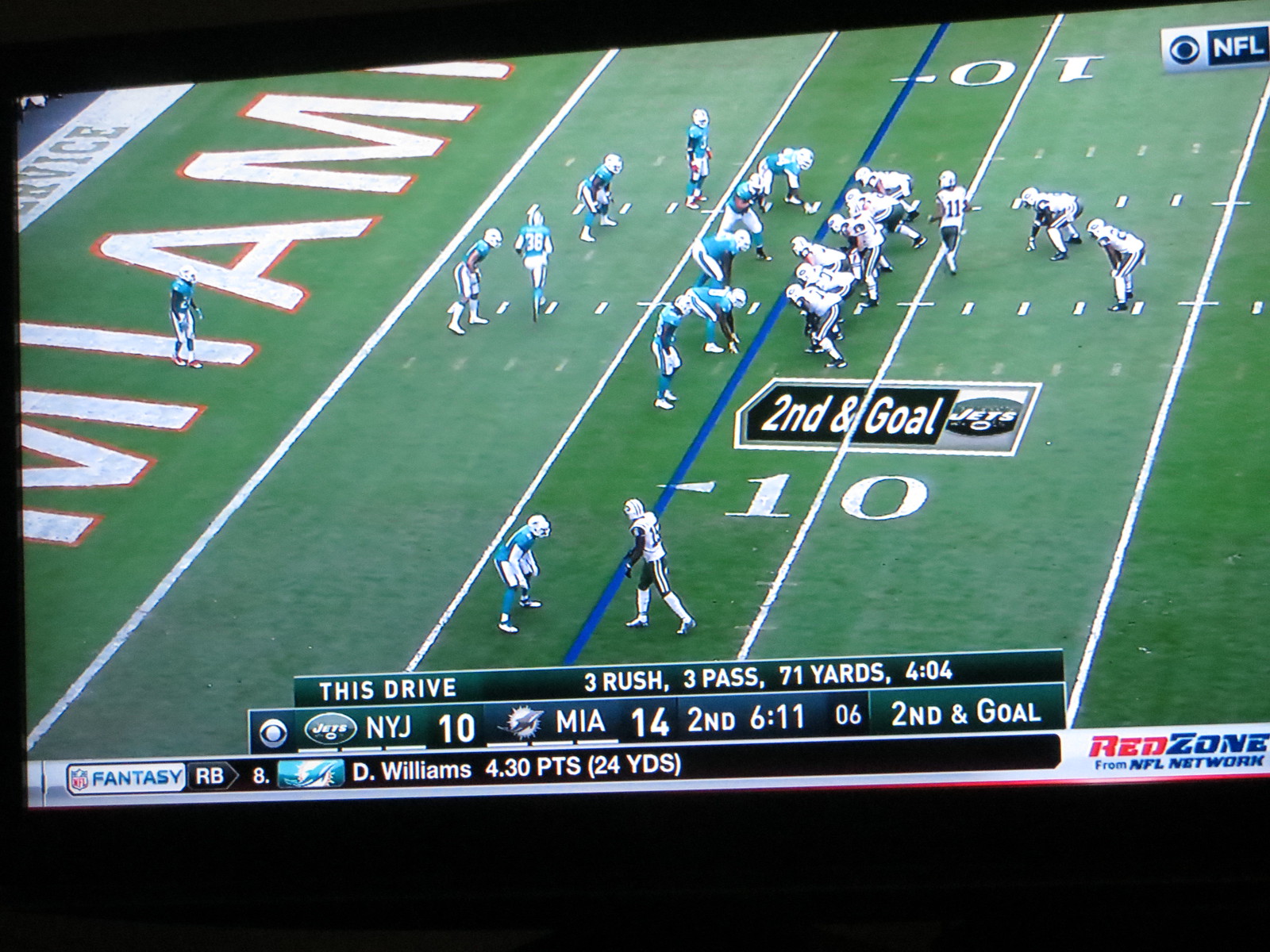The image depicts a slightly angled photograph of a flat-screen TV displaying a televised American football game. The TV screen exhibits a black background forming a long triangle at the top and a slightly less slanted black rectangle at the bottom. The football field displayed on the screen highlights the far end zone, prominently showing 'Miami' written in white letters with an orange border. The game features two teams, one dressed in blue and the other in white jerseys. The scoreboard indicates that the New York Jets, who have scored 10 points, are playing against Miami, which has 14 points. The scene captures a moment where it is second and goal, as noted in white text with a yellow arrow near the crowd of players. The players appear to be aligning themselves into formations, suggesting an imminent play, with some players positioned at the back of the lines. Additionally, the screen shows various game statistics, enhancing the broadcast’s informational aspect.